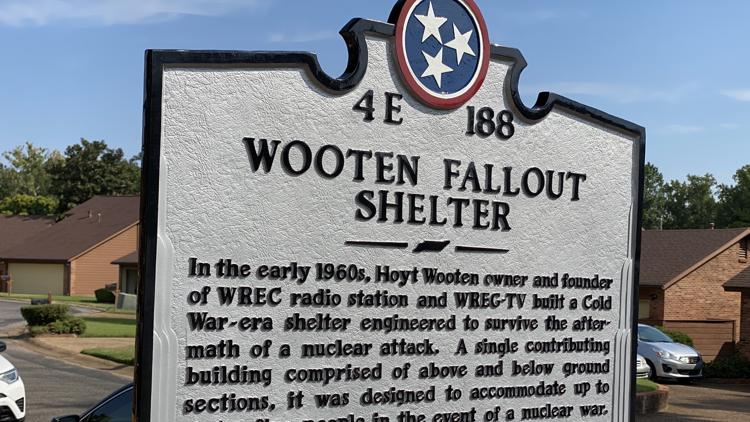This color photograph captures a metal sign, resembling a landmark plaque, situated in what appears to be a suburban subdivision. The background reveals a suburban street with single-story buildings, featuring brown roofs, brick and clavered facades, and an assortment of parked vehicles. The scene is set under a blue sky with scattered white clouds, accompanied by a line of green trees enhancing the backdrop.

The sign itself is predominantly white with a distinct black border at the top. Prominently displayed at the top of the sign is a circular emblem featuring a central blue circle adorned with three white stars, bordered by white and encased in a red outer ring. Below this emblem, the sign reads "4E188" in bold black text, followed by "Wooten Fallout Shelter" in large, striking letters. The lower portion of the sign contains smaller black raised text providing historical context: "In the early 1960s, Hoyt Wooten, owner and founder of WREC radio station and WREG-TV, built a Cold War era shelter engineered to survive the aftermath of a nuclear attack. A single contributing building comprised of above and below ground sections, it was designed to accommodate up to..." Unfortunately, the last part of the text is cut off and not visible in the photograph. This detailed sign offers insight into the historical significance of the fallout shelter and its Cold War roots, providing a glimpse into the measures taken during that tense period.